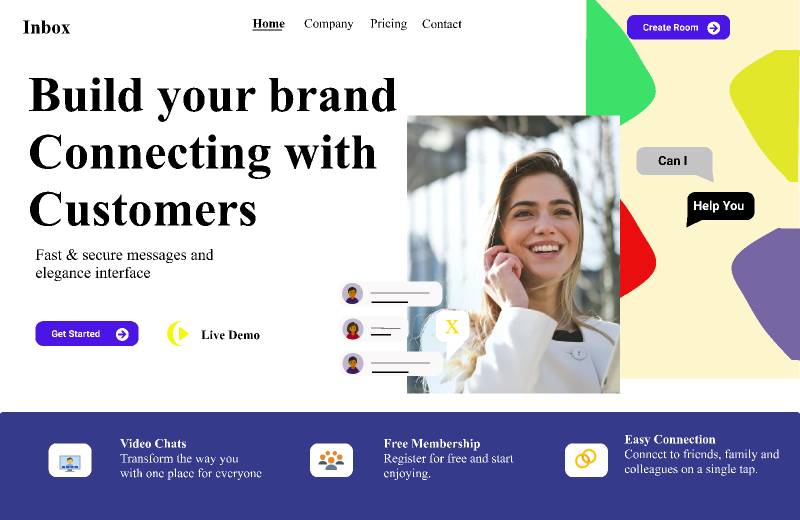This screenshot of a website prominently features a large, bold headline that reads "Build Your Brand Connecting with Customers." The main visual element is a photograph of a smiling woman wearing a white business jacket. At the bottom of the image, a dark blue banner is divided into three clickable sections, each with its own icon: "Video Chats," represented by a monitor icon; "Register for Free Membership," illustrated with symbols of people on cards; and "Easy Connection," denoted by two interconnected yellow circles. The top left corner of the screenshot displays the word "Inbox," while the top right corner features a clickable box labeled "Create a Room."